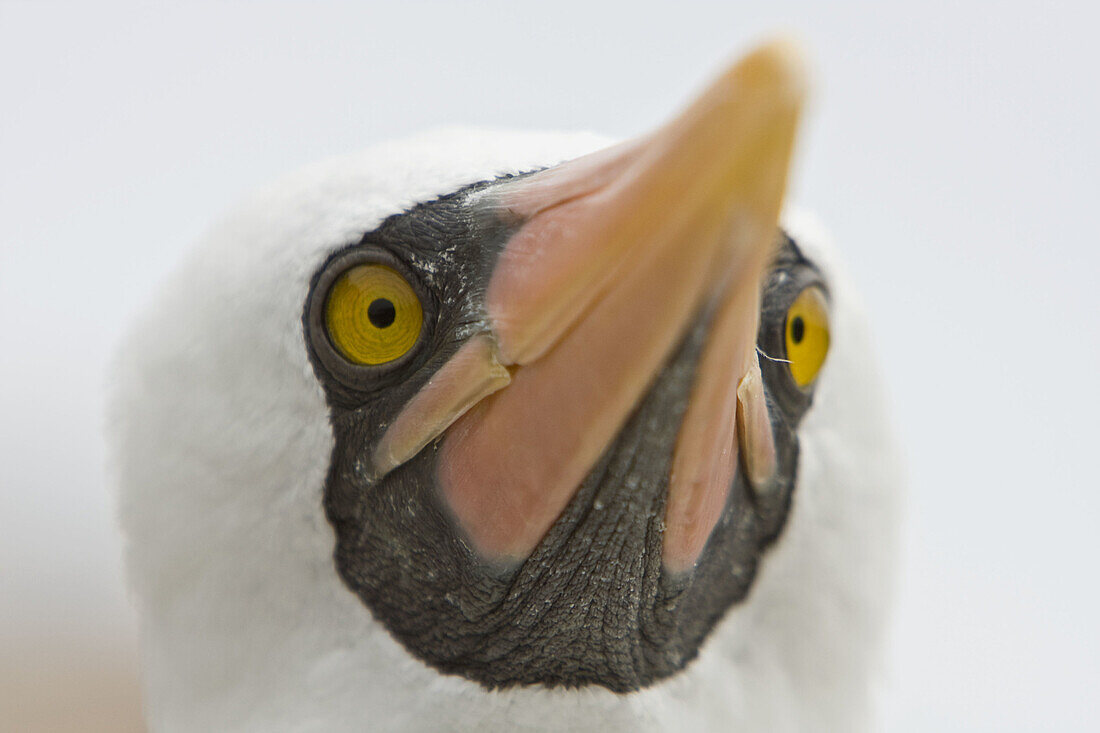This image showcases an extreme close-up of a bird's face, focusing from the neck up against a white background. The bird features predominantly white feathery hair surrounding its head, which gives it a round appearance. Its face, particularly around the eyes and towards the chin, reveals a black or dark gray-brown fleshy skin devoid of feathers. The bird has striking green eyes with black pupils that dominate the frame, appearing almost to stare directly at the viewer. Its peach-colored beak, transitioning from a pink tone at the bottom to a yellowish tone at the top, slightly juts upward towards the top right corner of the picture. The depth of field emphasizes the bird's eyes and head, while the beak, despite its detailed coloration, is slightly out of focus, adding to the dramatic intensity of the photograph.